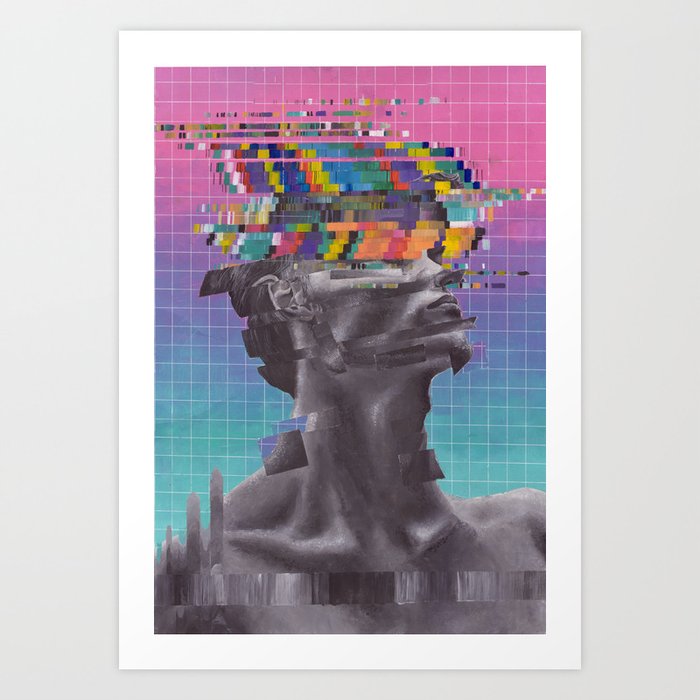This image features a meticulously designed poster with an overall gray background. Central to the composition is a white-bordered rectangle, which frames the main artwork. There's a noticeable grid of white horizontal and vertical lines providing structure across the poster. The background transitions from a vivid purple at the top to a darker purple, then to a deep blue, and finally to a light blue at the bottom. 

In the center of the image, a fragmented portrait of a man captures attention. His depiction spans from the top of his chest to the top of his head, with the face manipulated such that elements like his nose appear displaced, extending further than natural and creating a disjointed visual effect. At eye level and above, fragmentation intensifies, with his face dissolving into an array of colors and pixelated patterns. The area above his eyes is especially colorful, with lines in blue, pink, yellow, orange, purple, white, and turquoise, cascading horizontally and giving a sense of movement from right to left. The intricate interplay of colors and fragmented elements evokes a sense of digital manipulation, suggesting a transition or fragmentation of the subject within a digital context.